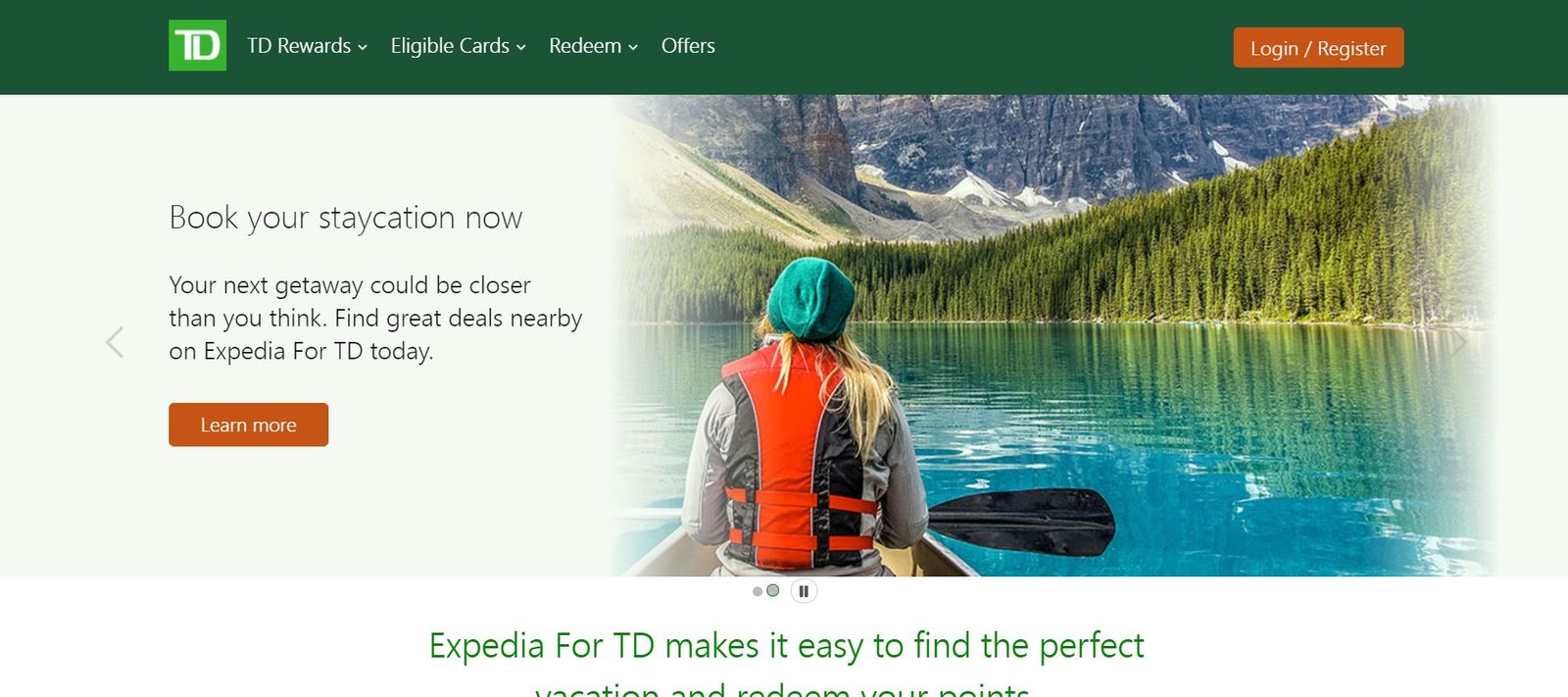This screenshot from the TD website or app showcases a user interface with a dark green banner at the top. On the left side of the banner is the TD logo, consisting of a light green square with the white letters "TD" in uppercase. The banner features several dropdown options labeled "TD Rewards," "Eligible Cards," "Redeem," and "Offers." Additionally, on the far right-hand side of this banner, there is an orange box with the text "Login Flash Register" in white.

Below the banner, on the right-hand side of the screen, there's a vibrant image of a woman kayaking or canoeing on a picturesque lake. She is wearing a life jacket and a blue-green beanie, surrounded by tranquil waters, lush trees, and majestic mountains, suggesting she might be in the Rocky Mountains, possibly near Banff or Lake Louise.

On the left-hand side of the image, there is a promotional text encouraging users to "Book your staycation now. Your next getaway could be closer than you think. Find great deals nearby on Expedia for TD today." A gray arrow points to the left, hinting at additional content. Below this text, an orange "Learn More" button invites further exploration. Underneath the image, partially visible green text states, "Expedia for TD makes it easy to find the perfect vacation and redeem your points," although the rest of the message is cut off, indicating that the screenshot does not capture the entire webpage.